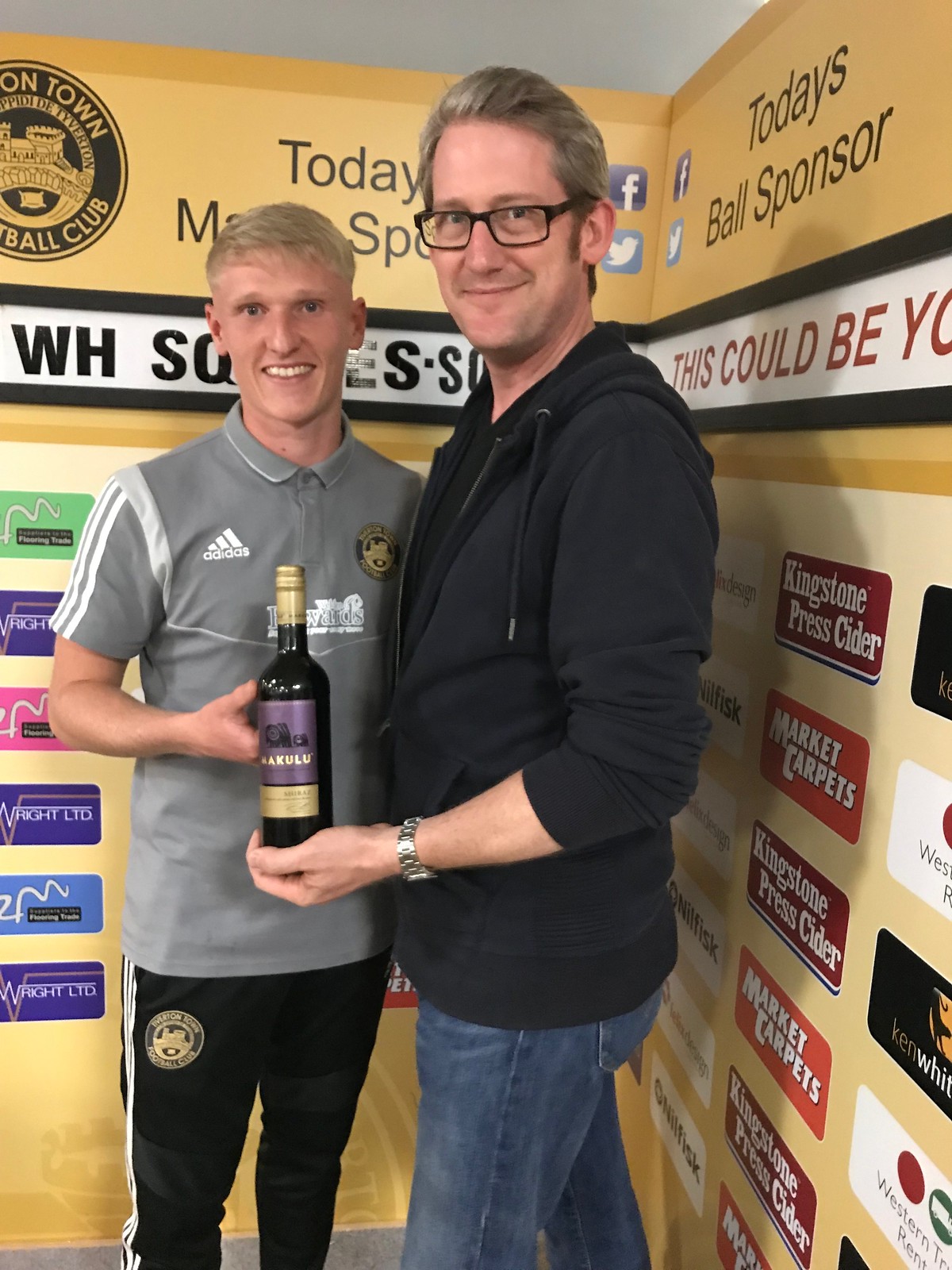The image features two men standing against a backdrop typically used for post-match interviews, adorned with numerous sponsor logos and banners. Prominent among these are Kingston Press Cider, Market Carpets, Wright Limited, and the Luton Town Football Club emblem. The backdrop also includes the text "Today's Ball Sponsors, This Could Be You."

The man on the left is dressed in sportswear that includes a grey Adidas shirt with white stripes along the arms, paired with black jogger pants that also feature white stripes and the Adidas logo. He has short blonde hair and is smiling, revealing his teeth.

The man on the right, noticeably taller, is wearing a black zip-up hoodie, blue jeans, and a wristwatch, and has black-framed glasses over his gray hair. He is tilting slightly to one side while holding a bottle of wine with a purple label and gold lettering that appears to read "Hakula" or "Kulu."

Both men are seemingly engaged in an informal photo, possibly taken in connection with a football event, considering the referenced Luton Town Football Club.